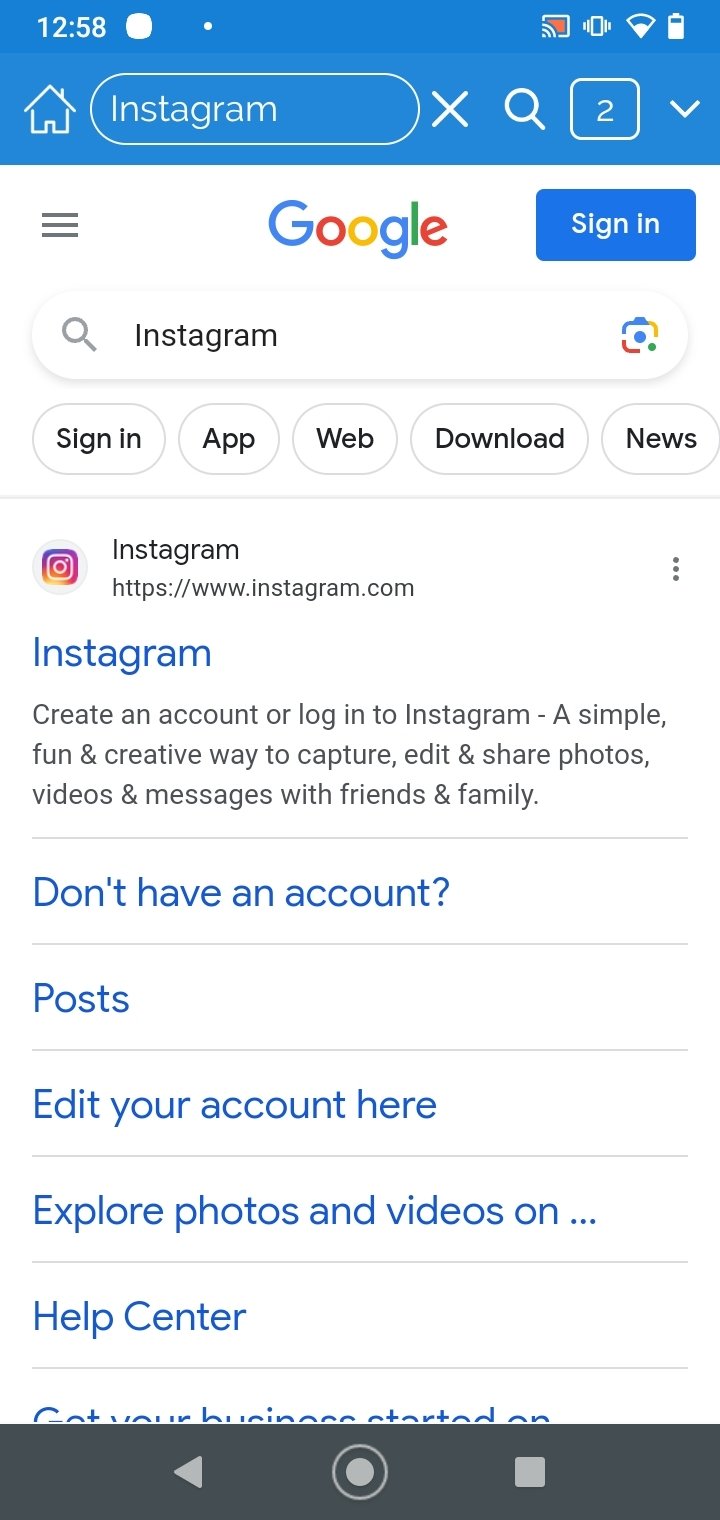The image is a screenshot of the Instagram webpage displayed on a computer screen. At the very top, there is a blue bar with white text and symbols. On the upper left-hand corner of this bar, the time "12:58" is displayed. Next to the time, there is an outline of a house icon in white, followed by a circular area with the word "Instagram" written in white inside the circle. 

Adjacent to this circle, there is a small "X" symbol, a search icon, and a white box containing the number "2." Above this blue bar, there are strength and battery icons typically found on a mobile interface.

Beneath the blue bar, the interface transitions to a white background. On the upper left side, there are three vertical black lines. Centrally displayed is the colorful Google logo, and next to it, a blue "Sign In" button. Below this, there is an Instagram search bar.

Further down, there are various options presented in small boxes labeled "Sign In," "App," "Web," "Download," and "News." Beneath this, the word "Instagram" is prominently displayed with the Instagram logo beside it.

Following this, there is a blue "Instagram" hyperlink with text inviting the user to create an account or log in, with a brief description stating: “A simple, fun, and creative way to capture, edit, and share photos, videos, and messages with family and friends.”

Below this, a series of blue links offer further options: "Don't have an account?" "Post and edit your account here," "Explore photos and videos on…" and "Help center." 

At the bottom of the page, partially obscured by a black bar, there is additional information. The black bar includes a left-pointing arrow on the left side, a central white button, and a white square on the right side.